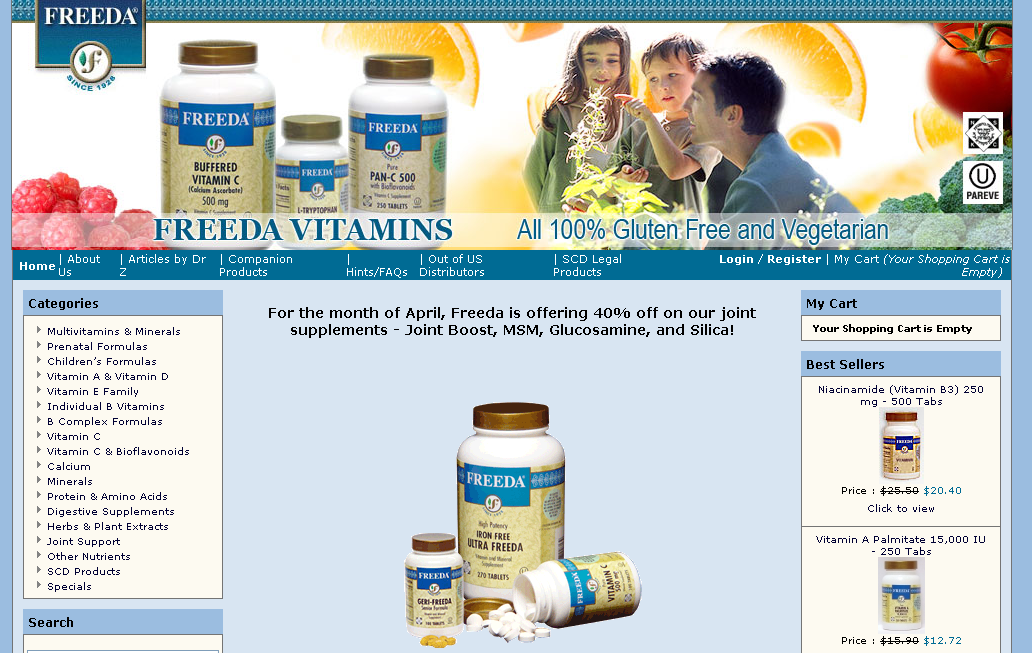This image is a screenshot of an online vitamin store. In the top left corner, there's a logo with a blue background, featuring the word "Freeda" spelled out as F-R-E-E-D-A, alongside a small "F" logo below it. Dominating the top third of the screen is a full-width banner image. This banner promotes "Freeda Vitamins," highlighting that all their products are 100% gluten-free and vegetarian. The image shows a scene with children and a father, possibly in a garden or park setting, looking at flowers, along with several vitamin bottles.

Directly below this image is a comprehensive menu bar stretching across the screen. The menu options listed include: Home, About Us, Articles by Dr. Z, Companion Products, Hints and FAQs, Out of U.S. Distributors, SCD Legal Products, Login/Register, and My Cart (noting that the shopping cart is currently empty in parentheses).

Underneath this menu bar, there is another section dedicated to product categories, featuring different types of vitamins such as multivitamins, vitamin C, joint support, and other nutrients. The central portion of the page displays some vitamin bottles, and on the right side, an empty shopping cart is shown. Below the empty cart, there is a list of best-selling products.

This detailed layout provides a clear and organized view of the vitamin store's offerings and functional areas.